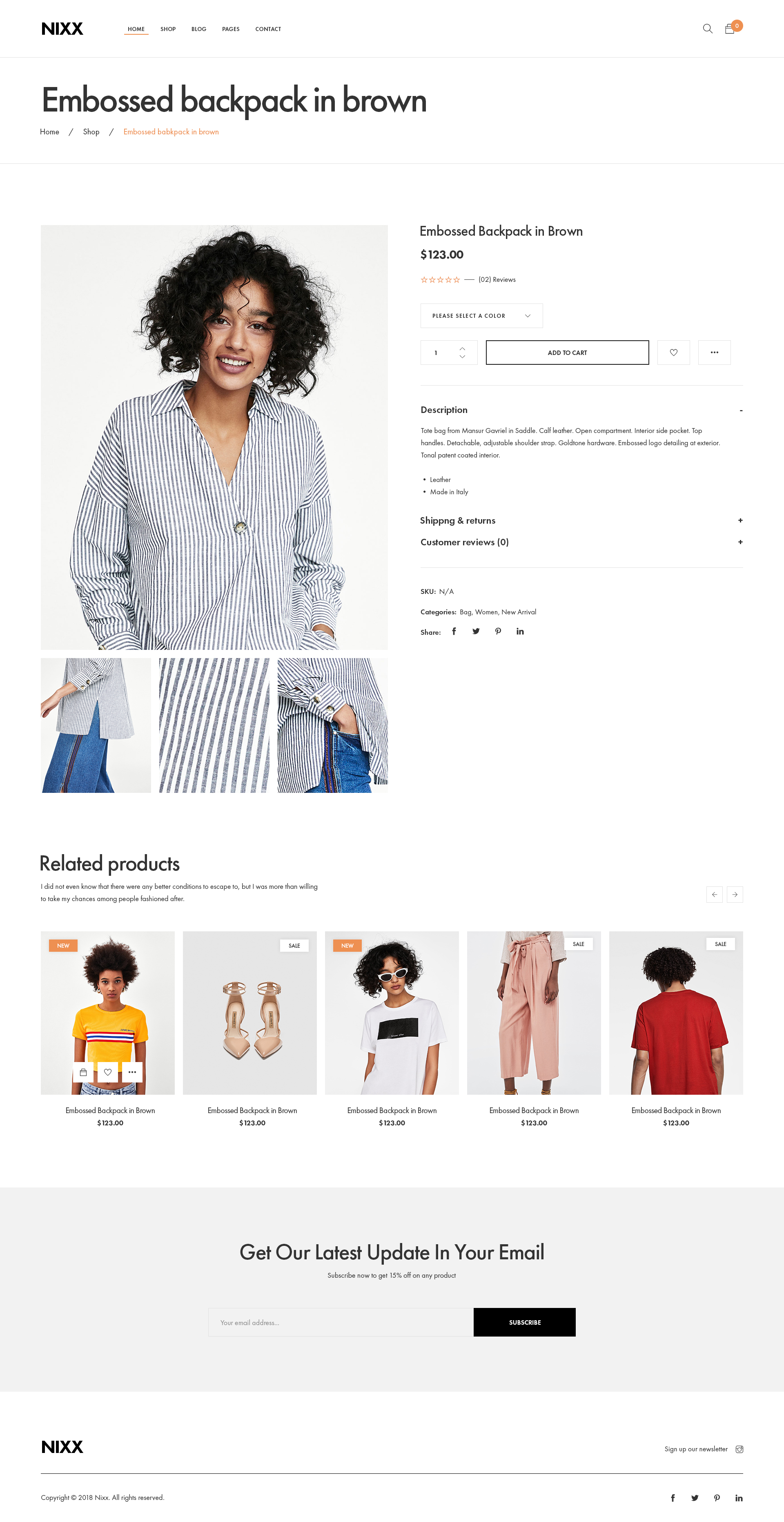This is an image of a website for women's clothing, named "Ni XX," with its logo located in the upper left corner. The navigation menu extends to the right with sections labeled: Home, Shop, Blog, Pages, and Contact. On the far right, there is an icon of a shopping bag with zero items and a search icon.

Currently, the website is on the Home page, indicated by a light brown underline beneath the word "Home." The main product highlighted on the page is labeled as "Embossed Backpack in Brown" priced at $123. However, the primary visual shows a long-sleeved, collared woman's blouse with blue and white stripes. Additionally, there are two reviews for the product, but no star ratings.

The product description mentioned, which should be for the blouse, instead describes a tote bag from the brand "Mons Min," made of saddle calf leather, featuring open compartments, an interior side pocket, top handles, a detachable adjustable shoulder strap, golden hardware, gold-tone hardware, embossed logo detailing on the exterior, and a tonal pattern with a coated interior. However, none of these details match the blouse shown in the image.